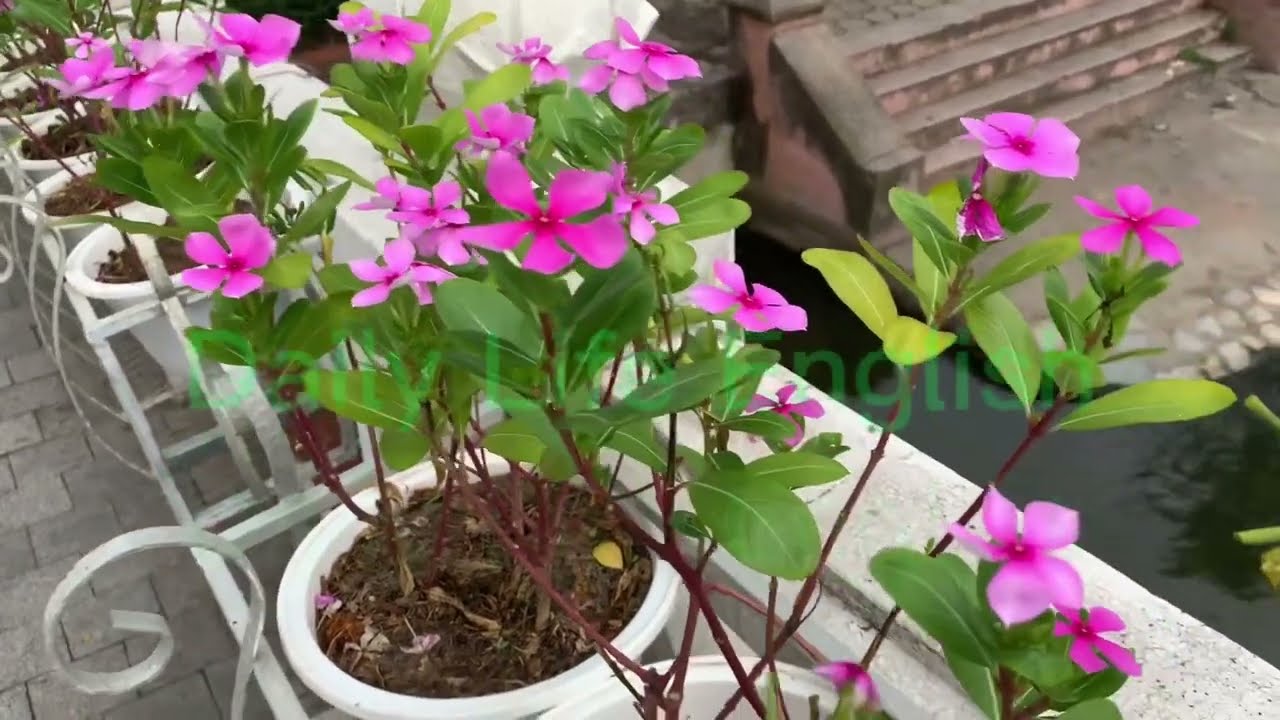This image depicts a wide, rectangular balcony adorned with a row of meticulously arranged potted plants. The balcony's edge, which extends from the bottom right corner to the top left corner, is constructed of gray, speckled concrete. The plants are housed in white pots secured within gray metal holders that line the entire edge of the balcony. The balcony floor consists of neatly laid gray bricks.

The plants, identified as Madagascar periwinkles, exhibit tall, delicate stems adorned with green leaves. The flowers themselves are pink, varying from light to darker shades and tend to have five petals each. The soil in each pot is a rich brown, contrasting with the clean white of the containers.

Beyond the balcony, a serene body of water is visible, its greenish hues reflective of the surroundings. In the top right corner, a gray concrete area with steps adds to the structural beauty of the scene, offering a glimpse into a larger patio space. There is a faint hint of some English text possibly written in green font, but it is difficult to decipher. The overall composition of the image combines the tranquility of nature with the orderly arrangement of the potted plants, creating a harmonious outdoor setting.